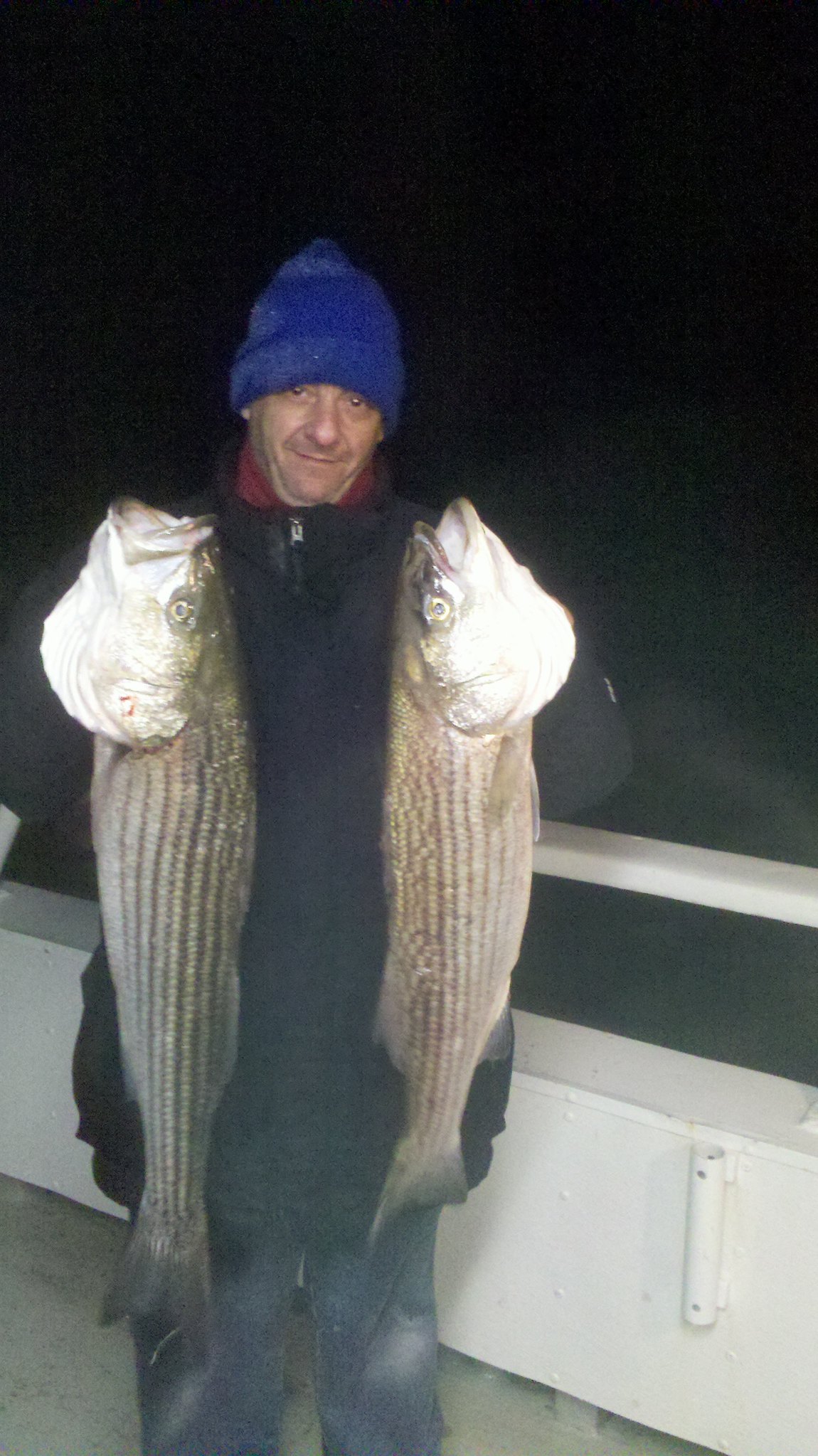In this nighttime photograph, a man stands centered in the image on a boat, holding two large, freshly caught fish by the gills. He looks directly at the camera, proudly displaying his catch. The man is dressed warmly, wearing a puffy black jacket over a red scarf, a blue shirt, blue jeans, and a red hat. A furry blue beanie caps his head. The boat's white guardrail and top frame the scene, while the bottom of the boat is gray. An empty fishing pole slot is visible below the railing, indicating the boat's purpose. The concrete-like floor beneath the boat hints at a sturdy construction. The colors visible include black, blue, maroon, tan, brown, green, and white, adding depth to the otherwise dark setting. There is no text in the image.